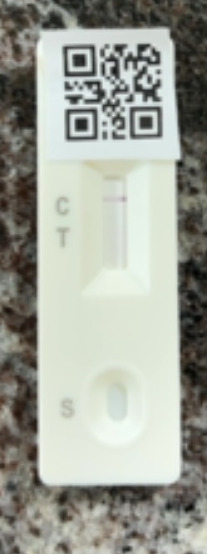The photograph depicts a COVID test kit lying on a speckled countertop, which appears to be a kitchen or work area surface characterized by a mixture of black, gray, and light-colored speckles. The background is slightly out of focus, directing attention to the test kit itself. The kit is off-white or light beige in color and prominently features a QR code sticker affixed at the top. Despite the general blurriness of the image, certain details of the test kit are discernible.

The COVID test indicator comprises several distinct areas: the 'C' (Control) and 'T' (Test) regions, which are recessed and shaped as vertical rectangles, and an oval-shaped sample application spot labeled 'S' at the bottom. Between the QR code sticker and the recessed indicator areas, a horizontal line is visible. No additional line is immediately apparent, though the blurriness of the image makes it difficult to determine if a faint second line exists. This might indicate a negative result, but due to the lack of clarity, a definitive interpretation cannot be made.